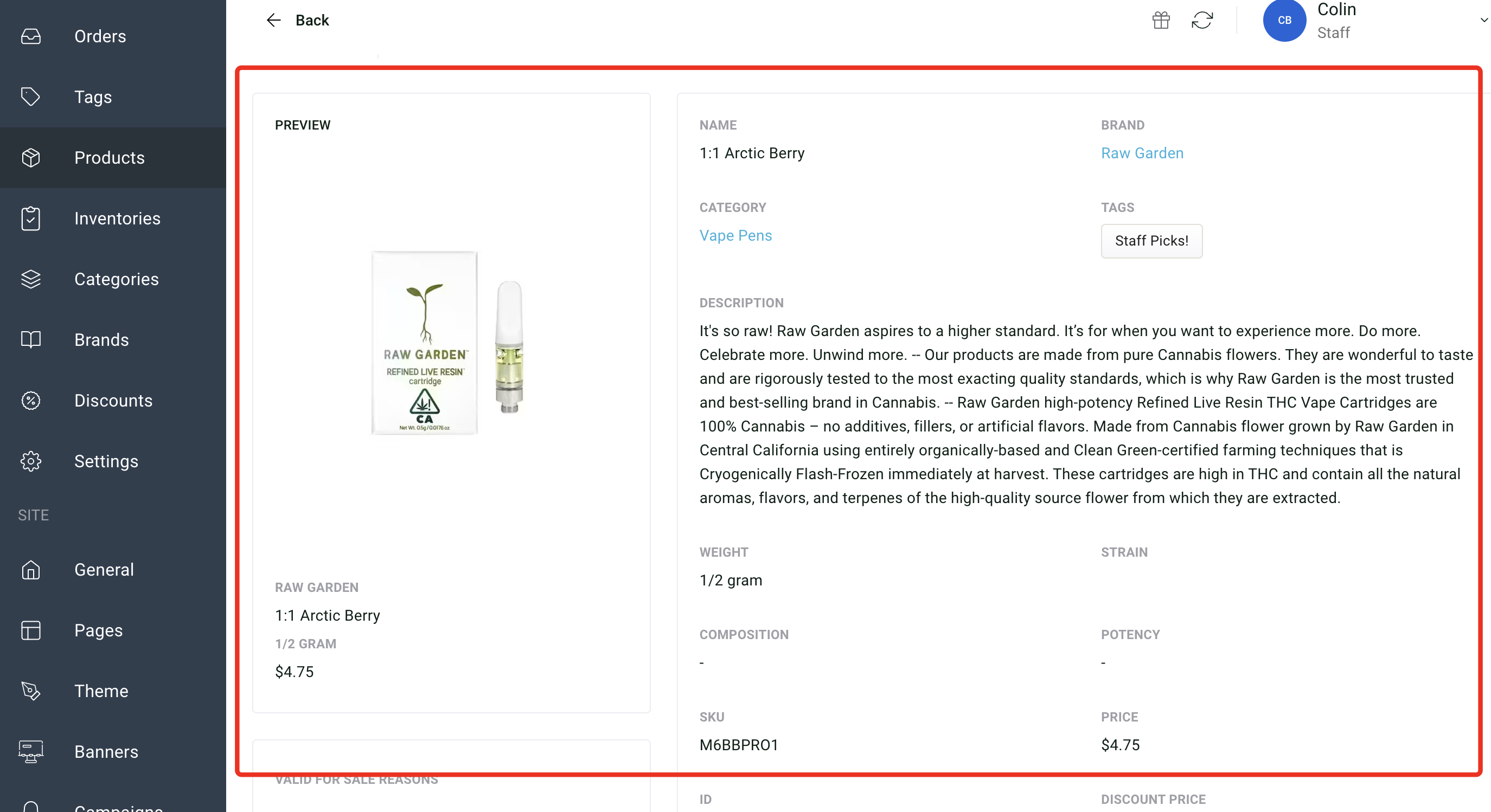The webpage is divided for administrative functions related to inventory management. 

On the left side, there is a vertical navigation bar with various tabs, each accompanied by small icons. The tabs include: Orders, Tags, Products, Inventories, Categories, Brands, Discounts, and Settings. Under the 'Site' section, additional tabs are listed: General, Pages, Themes, and Banners. 

At the top of the page, there is an option to navigate back, represented by a left-pointing arrow. To the right of this, there are several small icons, including one that appears to be a refresh symbol. Next to these icons, it shows the user status as "Collin Staff," with a small blue circle containing the initials "CE."

The main content area of the page displays detailed information about a specific product, likely a vaping product. Initially, there is a 'Preview' option followed by an image of a nozzle device. The product is titled "Salt Raw Garson Raw Garden" and specifics below it note: 

- "Raw Garden One-to-One Arctic Berry Half Gram" 
- Priced at $4.75.

More specific details are listed:

- **Name:** One-to-One Arctic Berry
- **Brand:** Raw Garden
- **Category:** Vape Pens
- **Tags:** Staff Picks

The description section contains an extensive text, presumably about the product. Below the description, various product specifications are listed but are partially incomplete:

- **Weight:** Half Gram
- **Strain:** (Not filled out)
- **Composition:** (Denoted by a dash)
- **Potency:** (Denoted by a dash)
- **SKU:** M6DBPRO1
- **Price:** $4.75